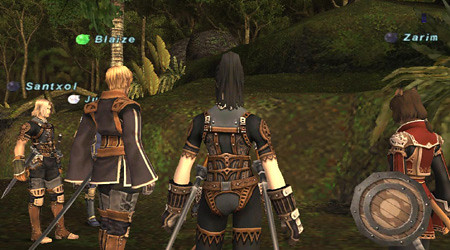In this image from a video game, we observe four figures, all clad in distinctive armor, with their backs turned toward us. Three characters have names displayed above their heads in blue letters: Zantzal is on the far left, Blaze is to their right, and Zareem stands on the far right. Zareem uniquely holds a shield.

Starting from the right, Zareem is dressed in red armor and has brown hair. Next to Zareem, the central character, lacking a name above their head, flaunts dark armor and dark hair, with two holstered swords on their back. To the left of this central figure stands Blaze, who sports elongated pieces of armor and blonde hair. Lastly, Zantzal, the figure on the far left, is outfitted in armor with short sleeves and also has blonde hair.

The backdrop features a serene landscape with lush green trees and grass, adding a natural contrast to the armored characters in this engaging video game still.